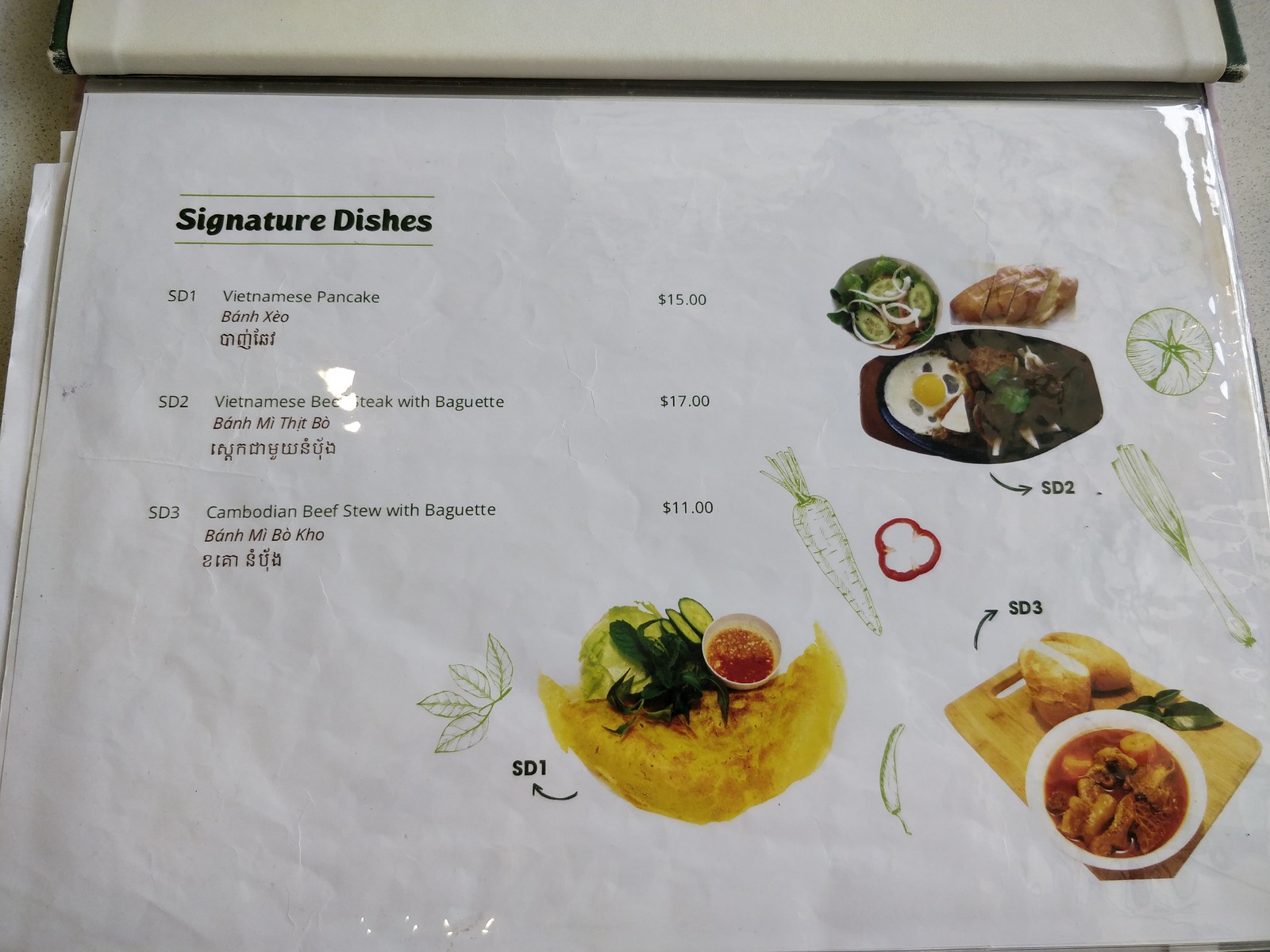The photograph showcases a page from a restaurant menu book. The menu is encased in clear plastic and laid on a white background speckled with subtle light gray dots. The binding of the menu book is folded back at the top, revealing green edges on both sides of the bent binding, with the central area of the binding appearing white.

The featured page is predominantly white and is titled "Signature Dishes" in the upper left corner, framed by two green lines—one above and one below the title. The offerings listed below the title include:
- Vietnamese Pancake, priced at $15.00
- Vietnamese Beef Steak with Baguette, priced at $17.00
- Cambodian Beef Stew with Baguette, priced at $11.00

Accompanying the text are photographs of the dishes positioned on the right and right-center portions of the menu. Additionally, the page is adorned with various green illustrations of vegetables and herbs, adding a decorative and thematic element to the menu design.